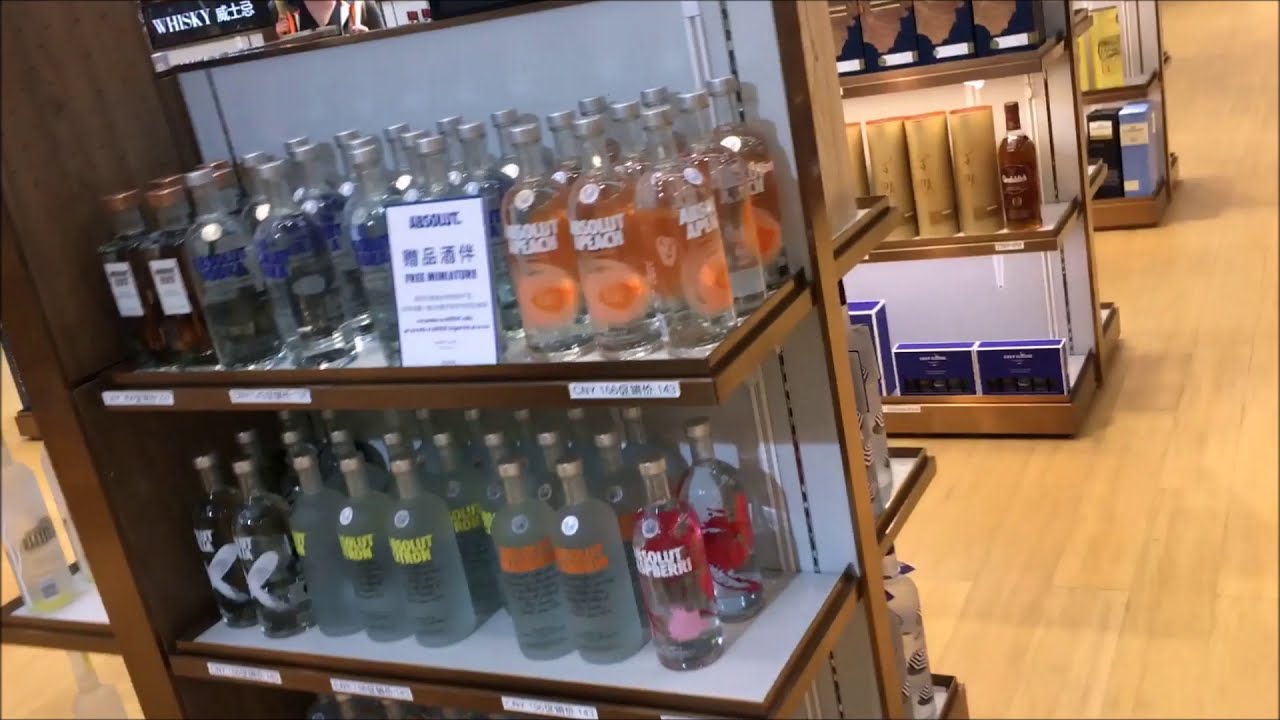The image depicts a tilted view of a well-organized liquor store, featuring modern shelving units with metal edges and white interiors, set against a light wooden floor. Prominently displayed in the foreground, a shelf is stocked with various flavors of Absolut Vodka, including Absolut Peach and Absolut Lemon, distributed across the top two rows. Behind this shelf, darker liquors like scotch or bourbon occupy the next shelving unit. Further back, a third shelf displays boxed bottles, the contents of which are not clearly visible. Signs and tags, some in English and some in an Asian language—possibly Korean or Japanese—suggest the store may be in an Asian country.